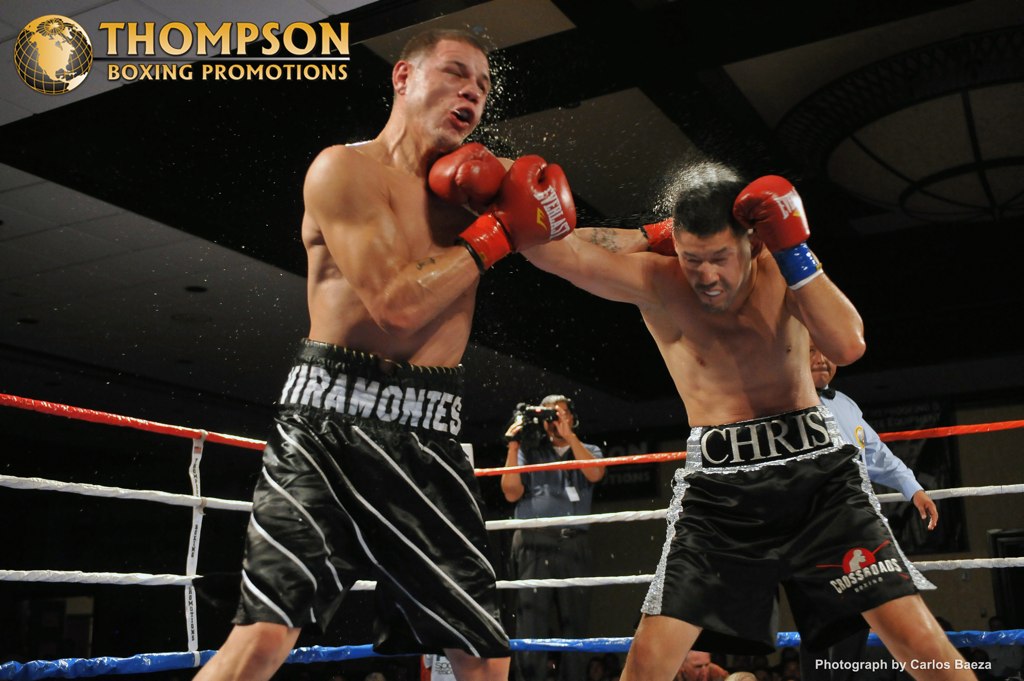The image captures a high-intensity moment during a boxing match. Both boxers are shirtless and clad in black pants. The fighter on the right, named Chris, is in the midst of landing a punch to his opponent's chin. He sports black pants with silver panels on the sides, and his name is emblazoned in light colors on his shorts. Chris has dark hair and appears to be wearing a white mouth guard, with his right hand up in a defensive position. His red boxing gloves feature blue near the wrists. The boxer on the left, whose shorts have white diagonal stripes and lettering that appears to spell Iremontes, is being struck in the face, causing his mouth to gape open. He has dark brown hair and is attempting to grab Chris's punching arm.

The action unfolds within a ring encircled by four ropes, colored red, white, white, and blue from top to bottom. Dark background tones accentuate the subject, and a cameraman dressed in blue and black can be seen capturing the fight. At the top left corner, the gold text "Thompson Boxing Promotions" is accompanied by a stylized gold globe. In the bottom right corner, the image is credited to "Photographed by Carlos Baeza."